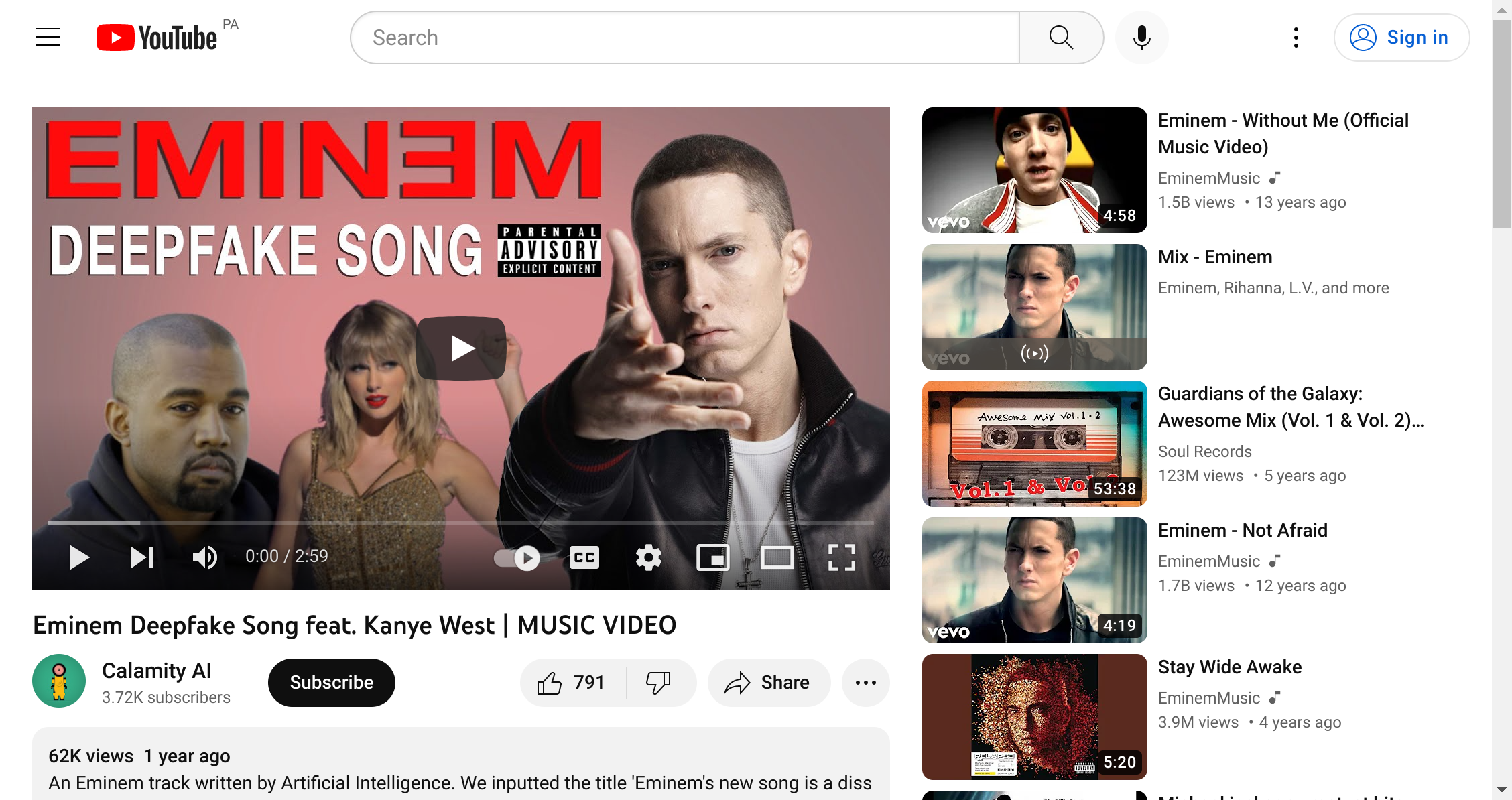The image depicts a YouTube interface with a white background. On the left-hand side, there are three horizontal black lines, indicative of a menu icon. To the right, there is a red rectangular box with a white play button triangle inside. Beside this box in bold black letters is the word "YouTube," and in the upper right-hand corner of this word, in smaller text, is "CPA."

At the top center of the image, there is an oval search box outlined in gray, with the word "Search" written in gray inside it, along with a gray magnifying lens icon on the right-hand side. Further to the right, a gray circle houses a black microphone icon. Adjacent to these, there are three black circles, followed by a gray and white background oval button that says "Sign In" in blue text.

Below the top navigation, a paused YouTube video is displayed. The video's play button is a white triangle centered on a black rectangle. At the top of this video, in red text, it says "Eminem." Beneath this, in white letters, it reads "Deep Fake Song," and there is a black and white "Parental Advisory Explicit Content" warning label.

To the right of the video preview, various artists are depicted: Eminem in the middle, Taylor Swift to the right, and Kanye West on the left. The video's description includes "Eminem Deep Fake Song featuring Kanye West," and the channel name appears as "Music Video Calling," which has 3.72 subscribers.